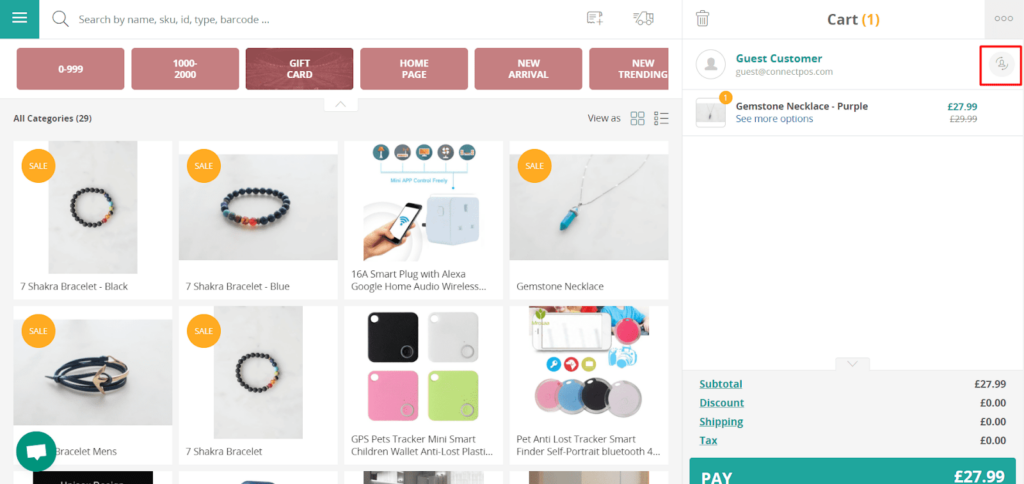This screenshot illustrates a shopping website interface, prominently featuring various navigational and functional elements. At the top, there is a search field capable of searching by name, SKU ID, or barcode. The navigation bar includes buttons labeled for item ranges "0 to 999" and "1000 to 2000," along with links to the gift card section, home page, newly arrived items, and trending products. On the right side of the top bar are icons for account management, the shopping cart, and additional options.

The main product display area showcases a diverse array of products organized in a grid layout under the category "All Categories (29)." Highlighted items include:
- A 7 Chakra bracelet in black, marked with a sale tag
- A 7 Chakra bracelet in blue, also on sale
- Another variant of the 7 Chakra bracelet with a sale tag
- A gemstone necklace
- A 16A smart plug compatible with Alexa and Google Home for audio wireless control
- A GPS-enabled Pet Tracker 
- A multi-functional Mini Smart Tracker suitable for children, wallets, and anti-loss purposes, equipped with Bluetooth technology. 

The interface is designed for ease of navigation and showcases a broad selection of items with clear, concise labeling and promotional tags on discounted products.